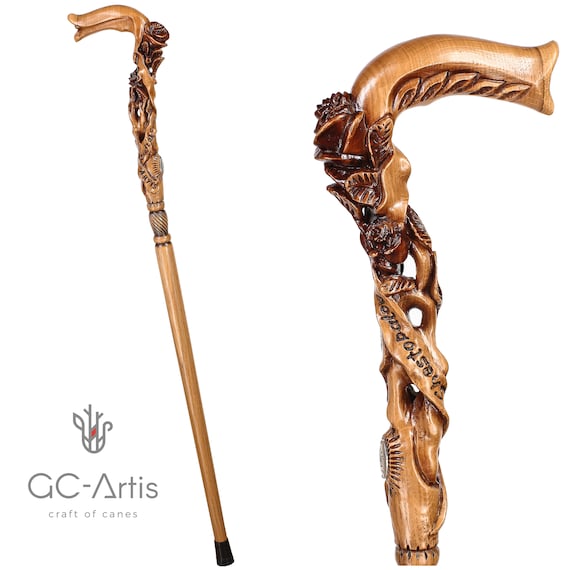The advertisement showcases an ornate walking cane crafted by GC Artists Craft of Canes. The ad features two distinct images of the cane: a full-length shot and a close-up detail. The cane, made from a light brown wood with a varnished sheen, exhibits a complex and elegant carved design that covers the upper portion. This intricate pattern, possibly inspired by flowers, leaves, and abstract shapes, twists and turns around the handle area. 

Additionally, the ad includes a logo depicting a stylized, pencil-drawn reindeer with antlers resembling tree branches and leaves, adding an artistic touch to the presentation. The background of the ad is entirely white, highlighting the craftsmanship of the cane. Latin inscriptions are visible within the design, adding to the cane's refined and superior aesthetic. This visually appealing presentation emphasizes the craftsmanship and artistic value of the cane, appealing to buyers interested in finely crafted walking sticks.